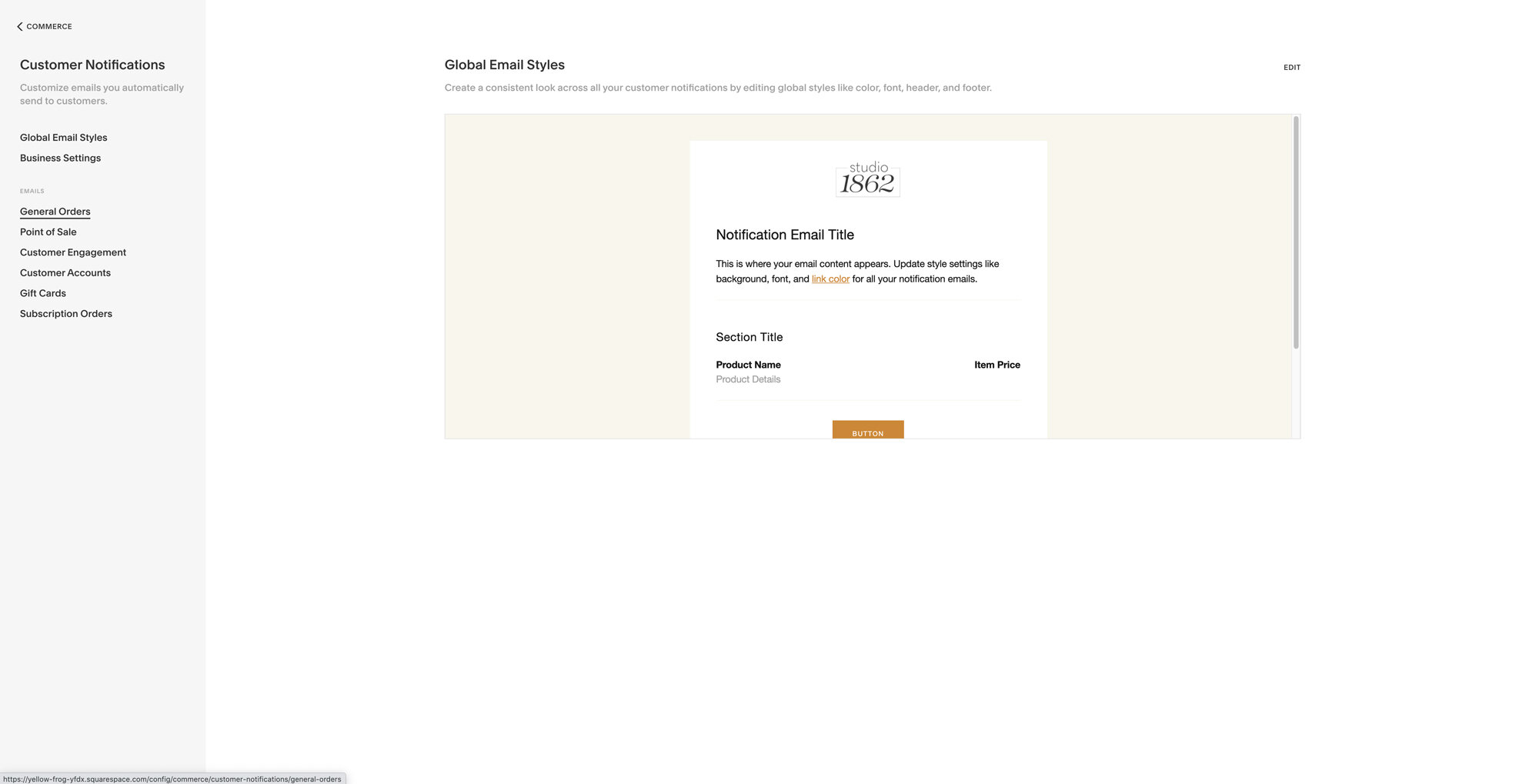The image on the left side displays a menu with various options related to customer notifications, including sections for customizing emails to be sent to customers, global email styles, business settings, and orders. Specific categories in the menu include General Orders, Point of Sale, Customer Engagement, Customer Accounts, Gift Cards, and Subscription Orders.

At the bottom left corner of the image, a URL is shown in detail: `https://yellow.flower.yafdx.square-space.com/config/commerce/customer-notifications/general-orders`.

In the center of the image, there's a highlighted section about setting a global email style. This feature allows the user to create a consistent appearance across all customer notifications by configuring the color, font, header, and footer. A tile labeled "Studio 1862 Notification Email" indicates the area where email content will appear, and it provides options to update style settings such as background color, font style, and link color for notification emails. The content includes sections tagged as Product Name, Product Details, and Item Price, accompanied by an orange rectangle button.

The center logo reading "Studio 1862" is displayed in an elegant cursive font. The background within the central window is gray, while the surrounding area is predominantly white space. A scrollbar is visible, and the top right corner of the screen contains an "Edit" option.